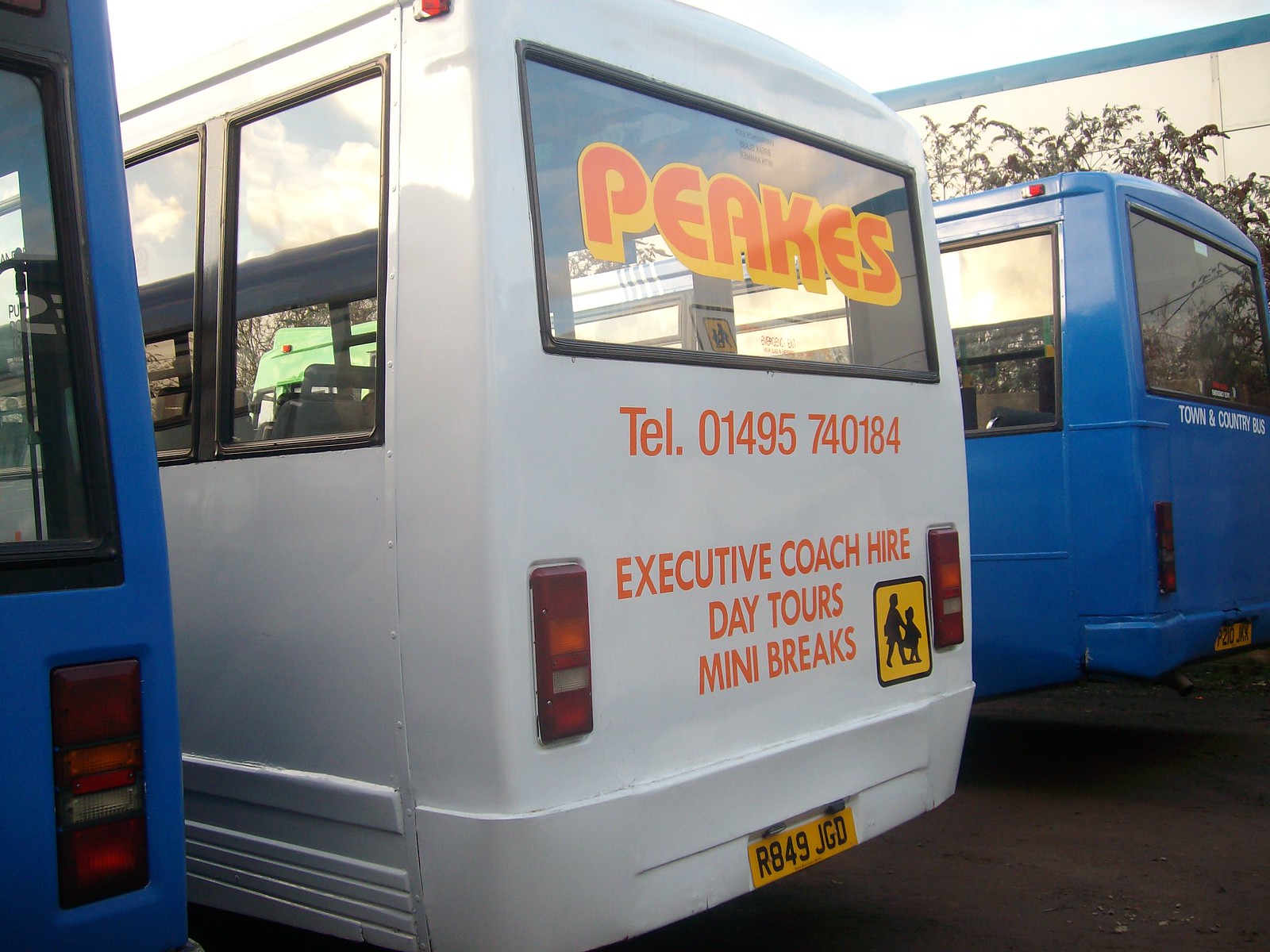This outdoor daytime photograph captures the rear ends of three parked buses positioned side by side, with their details sharply in focus. On the very left, a blue bus is partially visible, showcasing a bit of its window and one of its taillights. The bus in the middle, starkly white, prominently displays the text "PEAKS" in thick orange font with a yellow shadow, reminiscent of 1980s styling, across its back window. Additional information below this includes the telephone number "TEL 01495 740184" in a basic sans-serif font, followed by "Executive Coach Hire Day Tours Mini Breaks." A yellow traffic symbol depicting a person holding a child's hand appears on the lower right side of the bus. The middle bus also features a black-on-yellow license plate reading "R849JGD." On the far right stands another blue bus, adorned with the text "Town and Country Bus" in white below its rear window. The image's background includes a sky filled with clouds, a distant tree directly behind the rightmost bus, and a partial view of a building. Reflections of the clouds and surrounding scenery can be seen on the bus windows, adding depth to the composition.